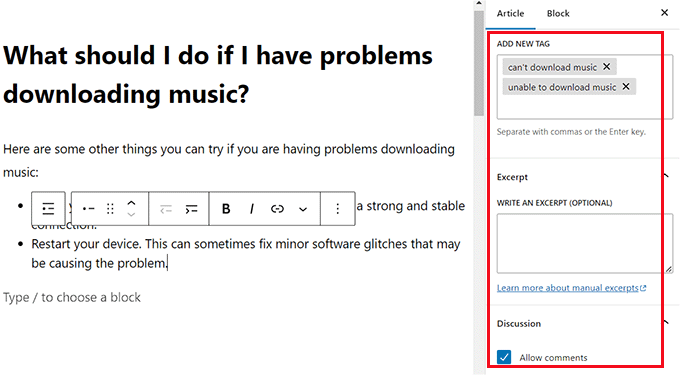The image depicts a screenshot of an instructional page dedicated to troubleshooting music download issues. The page is characterized by a white background with a bold, black heading at the top, stating, "What should I do if I have problems downloading music?" Beneath this, a subheading notes, "Here are some other things you can try if you're having problems downloading music."

Part of the text on the page is obscured by a formatting toolbar, featuring options such as alignment, italicizing, and hyperlinking. Following this toolbar, the visible text includes a suggestion to ensure "a strong and stable connection." Below this advice, another bullet point reads, "Restart your device. This can sometimes fix minor software glitches that may be causing the problem." 

Aligned to the left in gray text, there is an instruction, "Type / to choose a block."

On the right-hand side of the screen, a vertical menu is present. It has two tabs at the top labeled "Article" and "Block." The "Article" tab is underlined in blue, indicating it is currently selected. Within this section, there is an "Add New Tag" field, where two tags have been added: "can't download music" and "unable to download music," both displayed in gray. Below the tags field, there are instructions to "Separate with commas or the enter key."

Further down, an "Excerpt" section is present, encouraging the user to "Write an excerpt (optional)." A gray text box is provided for input, followed by a link titled "Learn more about manual excerpts."

At the bottom of the menu, a "Discussion" section includes a checkbox labeled "Allow comments," indicating that this option is selected.